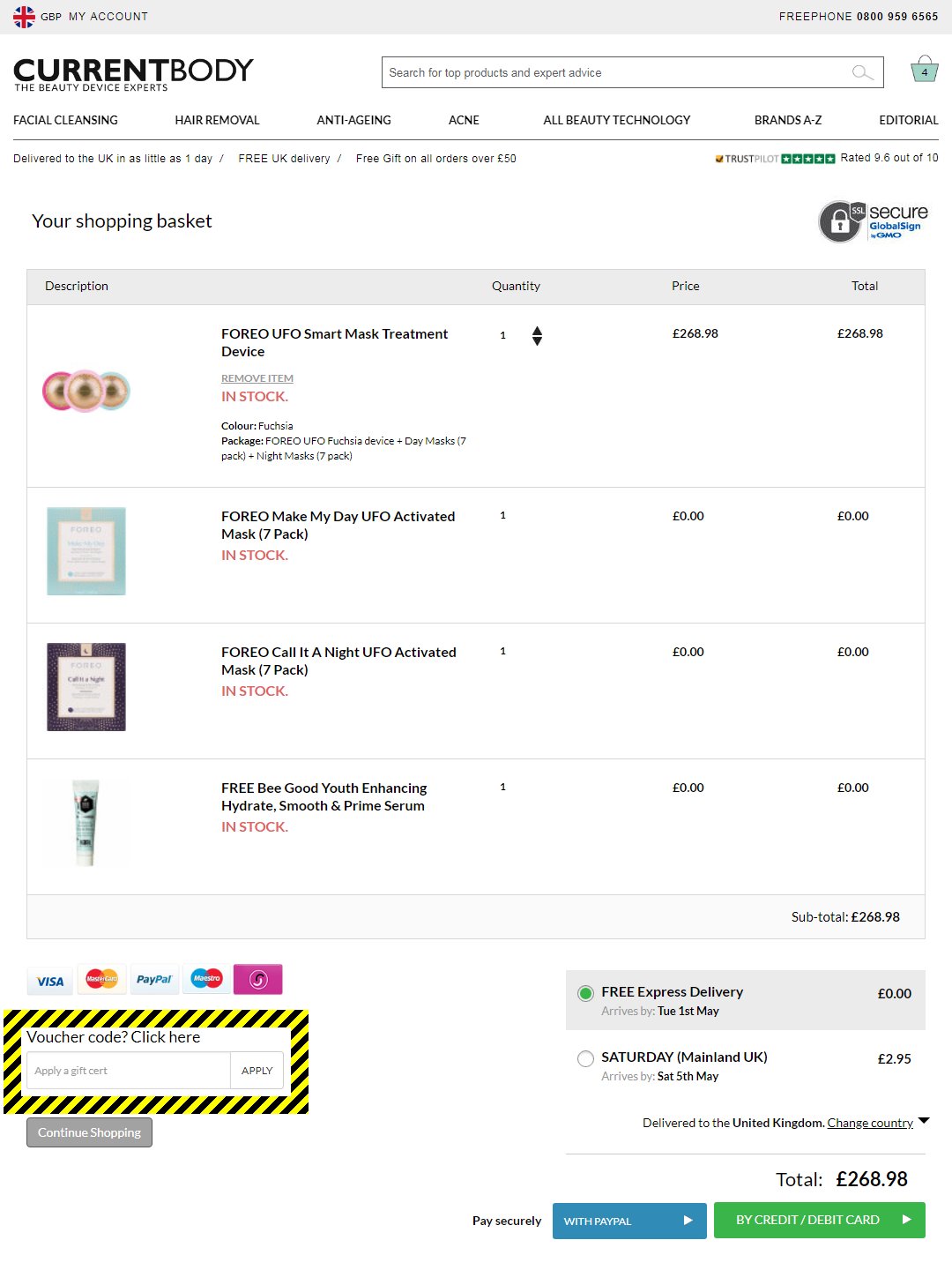The image is a screenshot from "Current Body: The Beauty Device Experts" website. The screenshot includes various sections such as "Facial Cleansing," "Hair Removal," "Anti-aging," "Acne," "All Beauty Technology Brands A–Z," and "Editorial." It highlights promotional text stating: "Delivered to the UK in as little as one day," "Free UK delivery," and "Free gift on all orders over £50."

The screenshot also shows a shopping cart containing four items:
1. Foreo UFO Smart Mask Treatment Device priced at £268.98.
2. Foreo Make My Day UFO Activated Mask 7-Pack with a price of £0.00.
3. Foreo Call It A Night UFO Activated Mask 7-Pack also priced at £0.00.
4. BeGlow Youth Enhancing Hydrate Smooth & Prime Serum offered for free.

Additionally, it mentions "Free Express Delivery arrives Tuesday, May 1st" at no extra cost. The total cost of the order amounts to £268.98. Payment options include PayPal or credit/debit card, and there is a circled prompt to "Click here" to enter a voucher code.

The user was likely providing details on how to get free shipping and promotional items by entering a specific code at checkout.